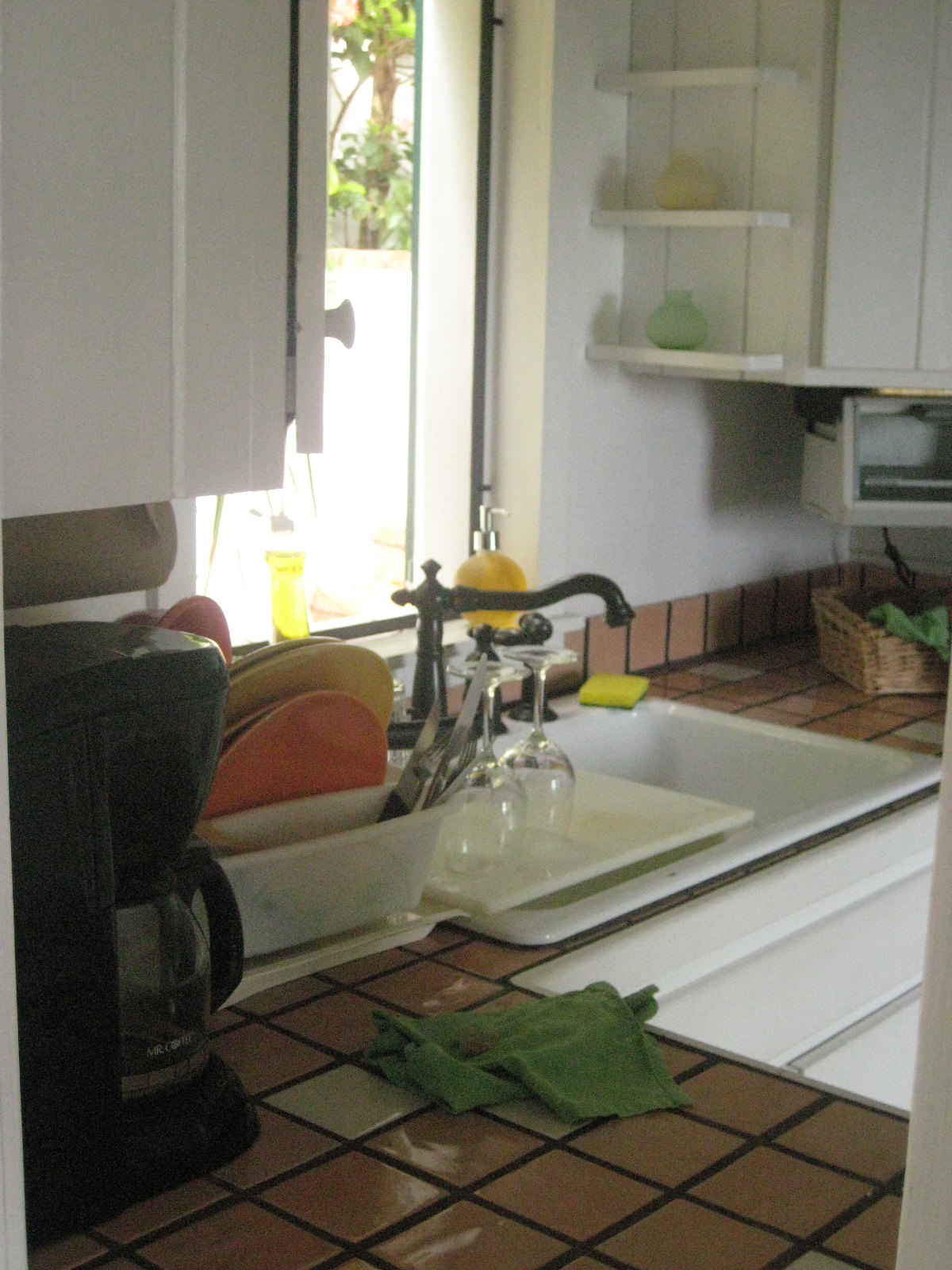This vibrant color photograph captures a cozy yet meticulously organized kitchen scene. The room, though relatively compact, exudes warmth and charm with its neat and tidy arrangement. The kitchen features ceramic tile countertops, which complement the white cabinets adorned with a classic beadboard design. The beadboard detail is also carried through to the area beneath the sink, enhancing the cohesive aesthetic.

At the heart of the kitchen, a white enamel or porcelain sink takes center stage, equipped with a pewter-finished faucet that extends gracefully over it. Directly above the sink, a window invites a flood of bright sunshine into the room, illuminating the space and offering a glimpse of a garden fence and greenery outside. A bottle of yellow dish soap sits conveniently on the windowsill, catching the light.

To the right of the sink, a small series of shelves provide both functionality and decoration. These shelves hold ornamental jars and perhaps a candle, all set against a backdrop of white beadboard. On the opposite side, to the left of the sink, two clear wine glasses rest on a rack or shelf, adding a touch of elegance. A coffee maker sits nearby, ready for use.

The countertop also displays a neatly arranged dish drainer, filled with freshly washed and stacked dishes, further emphasizing the kitchen's impeccable cleanliness. This photograph beautifully captures the essence of a well-kept, inviting kitchen bathed in natural sunlight.